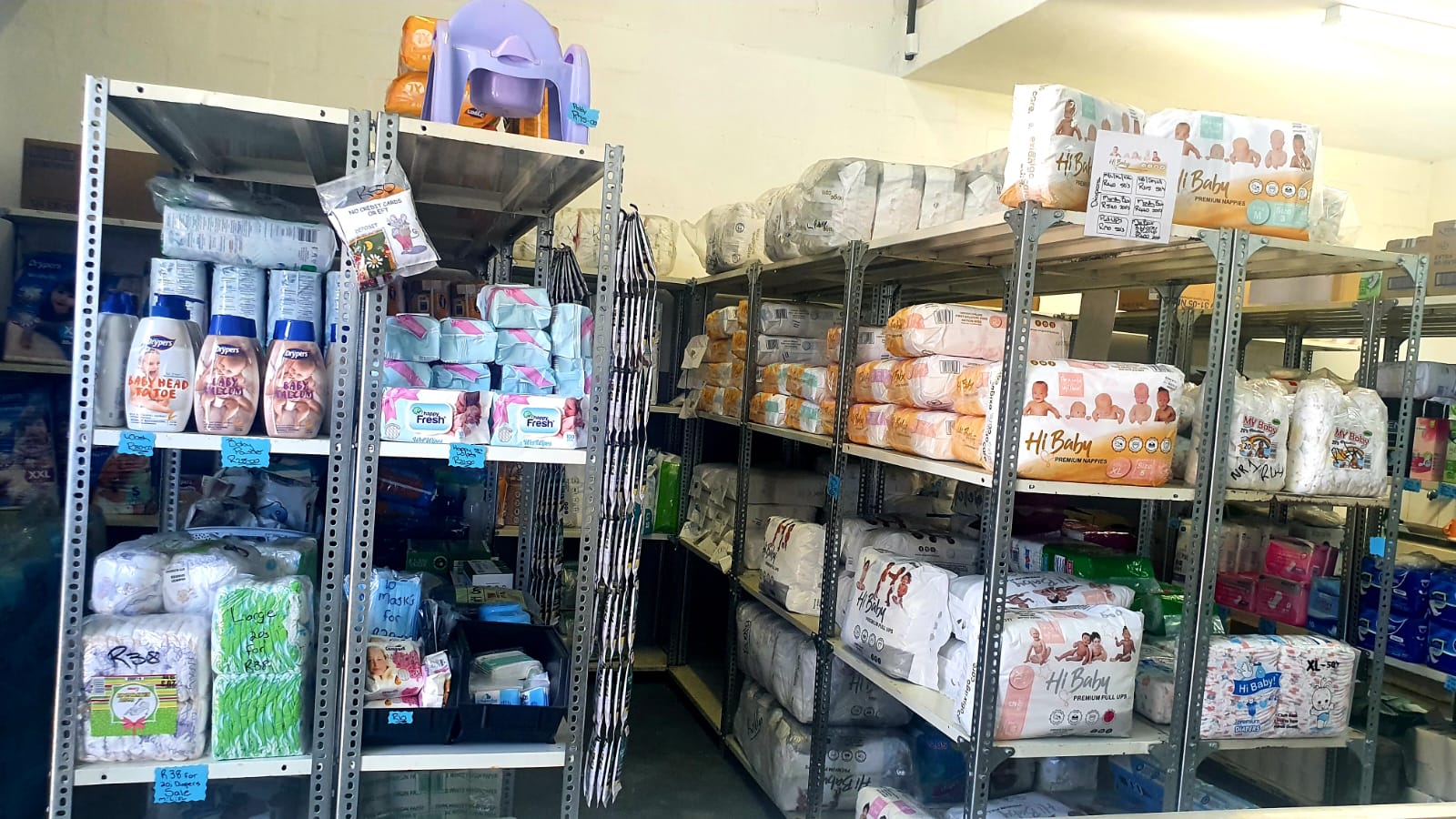The image depicts a storage area, likely a food pantry or a charitable distribution center, designed to assist individuals in need. The setting features large metal shelves stacked with various personal care items such as baby wipes, lotions, and other essentials on the left side. The floor is made of concrete, giving the area a utilitarian, warehouse-like feel. Adjacent to these shelves are rows filled with a wide assortment of diapers in various sizes and brands. The aisles between these shelves are narrow, allowing just enough space for a person to walk through comfortably. 

The atmosphere suggests that this is not a retail environment, as there are no price tags or commercial signs typically found in stores. Instead, handwritten signs are sporadically placed above the shelves, adding to the non-commercial ambiance. The shelves become even more tightly packed as one moves further into the area, necessitating sideways movement to navigate through them. The backdrop is characterized by drab, unadorned walls, further indicating that this is a functional space focused on aid distribution rather than consumer shopping.